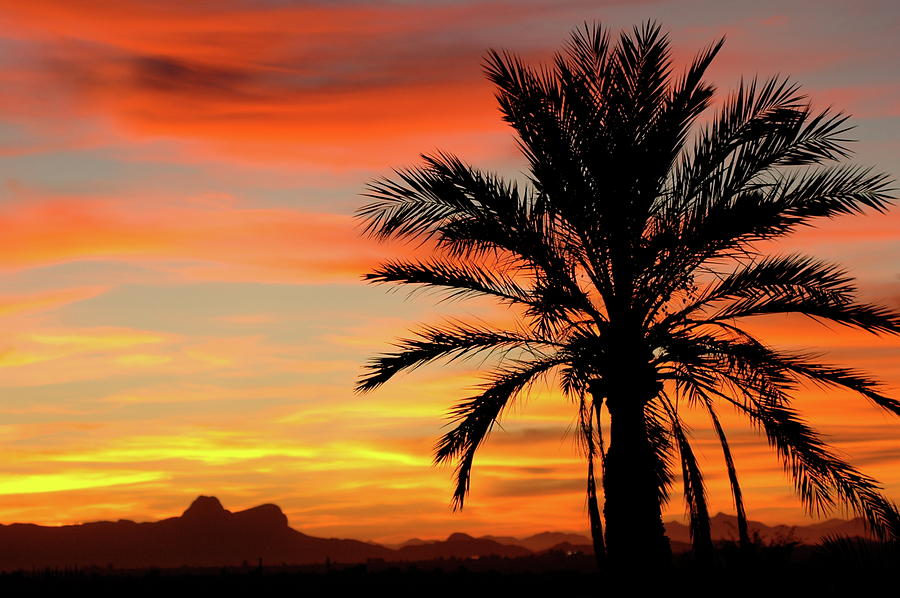The photograph showcases a striking silhouette of a towering palm tree set against a vivid and colorful sunset. The sky is ablaze with deep reds, fiery oranges, bright yellows, and soft peaches, blending into light blue and purple hues as it stretches upward. The palm tree, possibly a large date palm, stands prominent with its numerous fronds splayed out, casting a dramatic black shadow. The scene is further enriched by the presence of distant rounded hills or low-level mountains, their steep, ancient ridges barely perceptible in the fading light. The lower portion of the landscape also features hints of other trees and foliage, adding depth to the serene vista. The overall composition underscores the interplay of light and shadow, capturing the ephemeral beauty of the moment just before the sun fully sets.